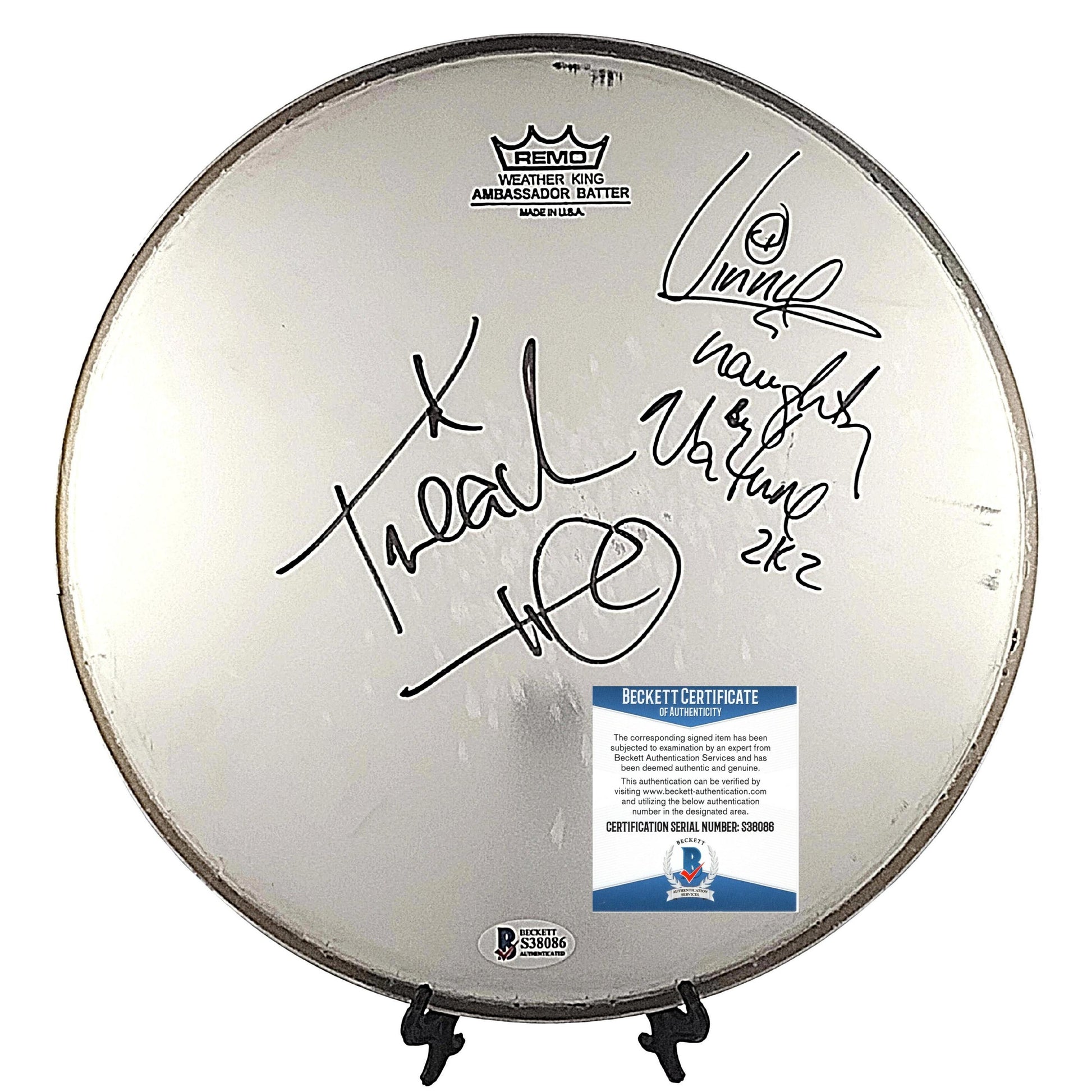The image features a round metal disc, prominently autographed and displayed upright on a black stand. At the top of the disc, a logo reads, "Remo Weather King Ambassador Batter, Made in USA," indicating the likely manufacturer and model. At the bottom, another logo states, "Beckett S38086 Authenticated," alongside a "B" check mark symbol. The center of the disc showcases an illegible cursive autograph. Also affixed to the disc is a large square sticker that details the Beckett Certificate of Authenticity. This sticker explains that the signed item has undergone expert examination by Beckett Authentication Services and is deemed authentic. Verification of the authentication can be performed by visiting www.beckettauthentication.com using the provided authentication number. The colors in the image predominantly include blacks, whites, grays, with accents of blue, grayish brown, and red, making the entire piece visually cohesive while adding to its authenticated charm.